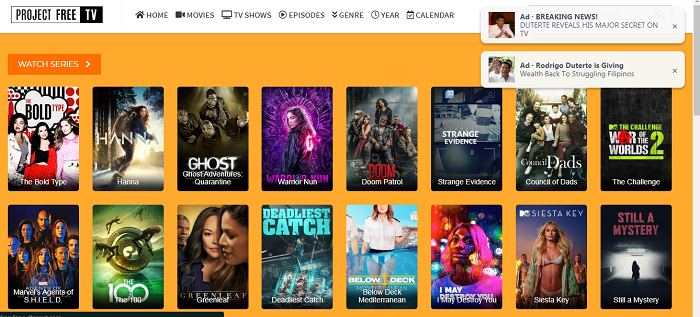The image is a vibrant, colorful screenshot of a webpage from Project Free TV, featuring a yellow and orange background with various TV show depictions. The top of the page displays the "Project Free TV" logo in bold black and white font set against a white background. Below the logo, the navigation bar includes icons and text for several sections: "Home" with a house graphic, "Movies" with a film reel graphic, "TV Shows" with a television graphic, "Episodes" with a play button, "Genre" with two downward arrows, "Year" with a clock, and "Calendar" with a calendar icon. 

Above the main content, breaking news headlines stand out against the page—highlighted ads announce, "Ad: Breaking News: Duterte Reveals His Major Secret on TV" and another noting, "Ad: Rodrigo Duterte is Giving Wealth Back to Struggling Filipinos."

The main section of the webpage features colorful thumbnails representing different TV shows. "The Bold Type" is depicted with an image of three women, "Deadliest Catch" with an action shot of a fishing boat, "Below Deck Mediterranean" featuring a stewardess holding a tray, and "Siesta Key" showing a young woman in a bikini.